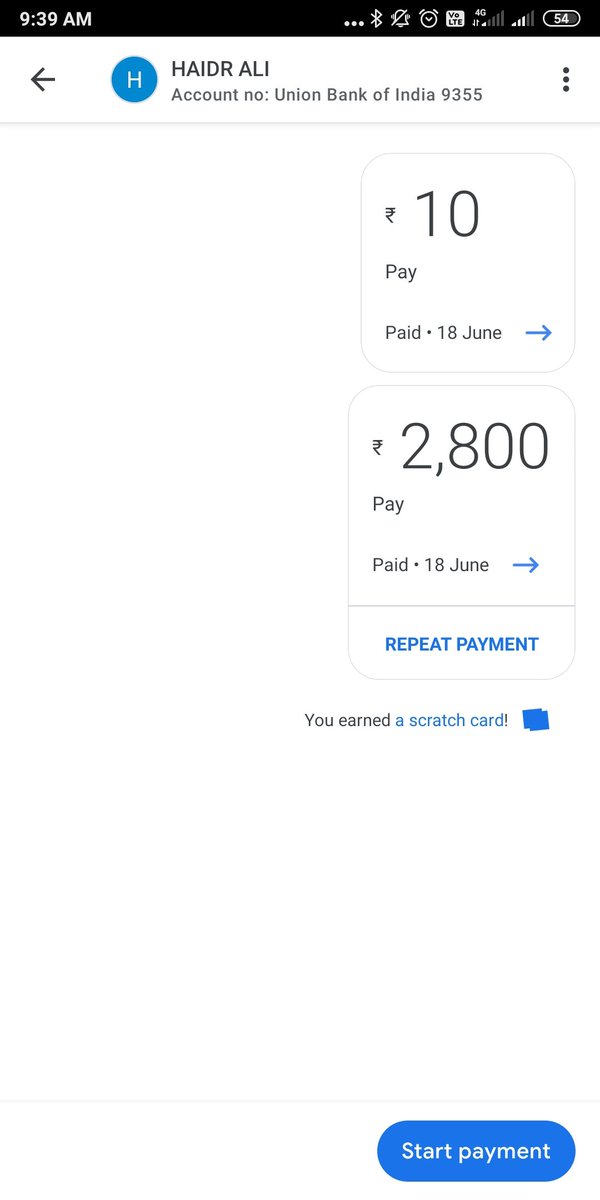This image is a detailed screenshot from a smartphone with a white background. The header at the top is black, displaying key information. On the left side, in white font, the time is shown as 9:39 a.m. On the right side, icons indicate the battery level at 54%, the 4G wireless network status, an alarm clock, and a notification bell.

Directly beneath the header, against the white background, there is a blue oval with a turquoise hue featuring a white letter "H." To its right, it says "HAIDRA ALI." Below this, the text specifies "Account Number," followed by "Union Bank of India 9355."

To the right, there's a vertical rectangle showcasing the word "Pay" with the number "10" above it and "Paid 18 June" below. Further down, the number "2,800" is displayed prominently, followed by "Pay" and "Paid 18 June." In blue font beneath this section, it reads, "Repeat Payment."

At the bottom right-hand corner of the screen, there is a blue button in the shape of a rectangle with rounded corners, featuring the text "Start Payment" in white. Additionally, near the bottom, there is a message indicating, "You earned a scratch card!" with an exclamation mark.